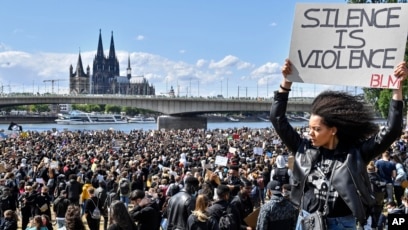In this detailed landscape photograph taken by the Associated Press, we see the vibrant scene of a Black Lives Matter protest on a sunny day with blue skies and scattered white clouds. In the foreground, a woman in a black leather coat holds a prominently displayed sign that reads, "Silence is Violence," with "BLM" inscribed in red at the bottom right corner, signifying the Black Lives Matter movement. Surrounding her is a massive, peaceful crowd of thousands, all gathered in what appears to be a park along a riverbank. The river is spanned by a wide, concrete auto bridge in the background, with docks and sailboats visible on the far side. Dominating the distant horizon is an imposing castle-like structure or cathedral with multiple spires, adding a dramatic architectural element to the scene. The photograph captures a powerful moment of solidarity and protest, underscored by the serene yet striking backdrop.